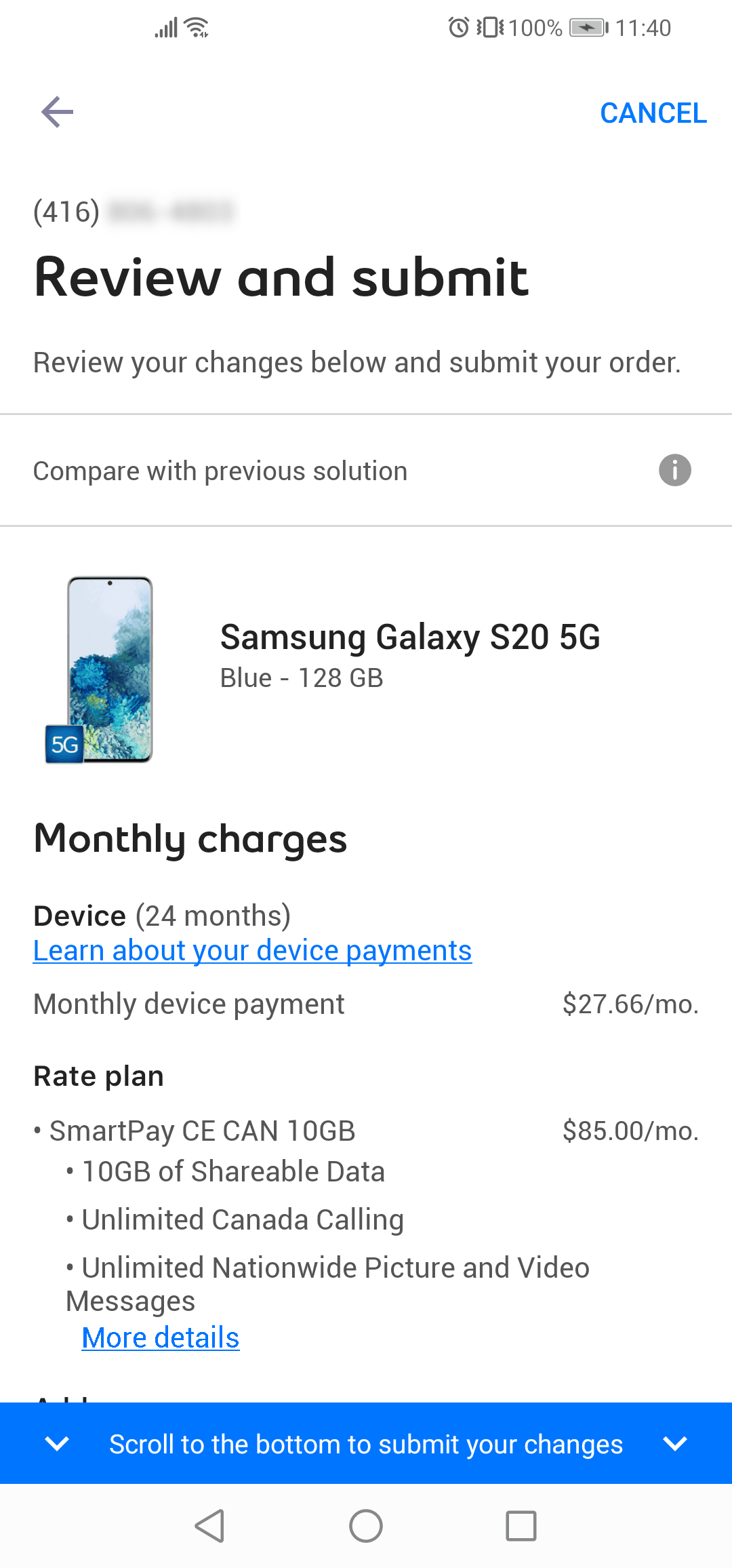This vertical image features a smartphone screenshot with a white background, likely captured from a device's screen. Starting from the top left, the status bar displays the signal strength icon and Wi-Fi icon, indicating connectivity. On the right side, the clock shows the time as 11:40, the battery icon is fully charged at 100%, and the device is currently charging.

Beneath the status bar, there is a back arrow on the left, and on the opposite side, highlighted in blue, is the "Cancel" option. Below this header, in bold text, it reads "Review and Submit" followed by instructions: "Review your charges below and submit your order." 

A horizontal line divides this section from the next, which has the text "Compare with previous solution" alongside a gray circle containing a white information 'i' icon.

Further down, the device details are listed:
- Samsung Galaxy S20 5G Blue
- 128 gigabytes

An image of the phone is displayed, followed by an itemized breakdown of monthly charges, including device cost and rate plan. The page concludes with a prominent blue button prompting users to "Scroll to the bottom to submit your changes."